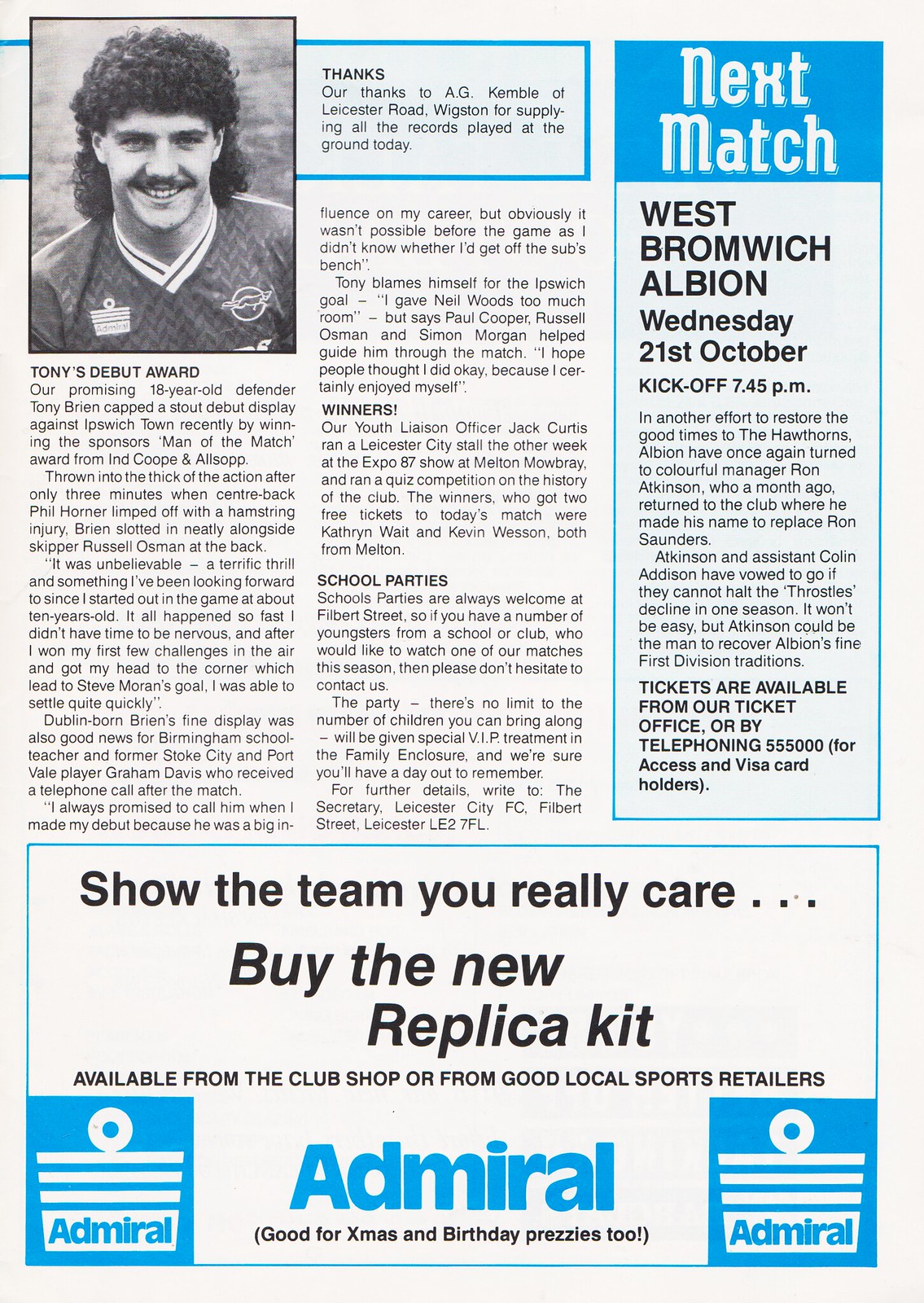This appears to be a vintage page from a magazine, featuring a black-and-white image of a football player in the upper left-hand corner. The player, identified as Tony Breen, an 18-year-old defender, sports long curly hair, a mustache, and a sports jersey. The caption under his photo announces his commendable debut, where he won the sponsor's Man of the Match award in a game against Ipswich Town, credited to A.G. Kimball of Leicester Road, Wigston, for providing the records played at the ground. The page also has an article titled "White on Blue, Next Match" in a blue frame on the upper right, detailing an upcoming match against West Bromwich Albion on Wednesday, 21st October, with kickoff at 7.45 p.m., and where to get tickets. At the bottom is a prominently framed advertisement from Admiral, a sports retailer, urging fans to "Show the team you really care; buy the new replica kit," available from the club shop or good local retailers, described as ideal for Christmas and birthday presents. The overall layout and content, paired with the vintage appearance and style of the player's photograph, suggest this page dates back to the 1970s.